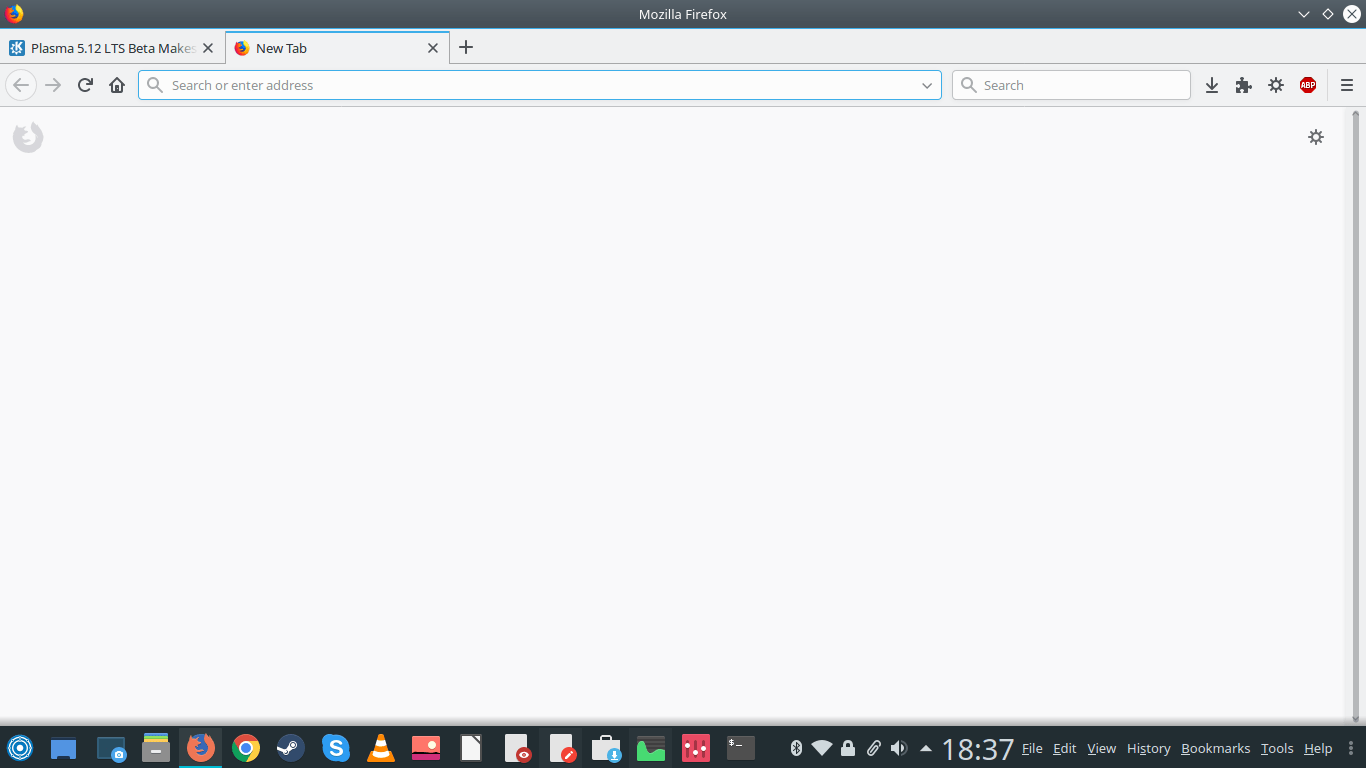This is a vertically-oriented screenshot of a website, captured from a laptop or computer. The image features distinctive elements of the Mozilla Firefox browser interface. Across the top of the screenshot is a dark grayish-black border featuring the text "Mozilla Firefox" in white, centrally positioned. On the upper left-hand corner, the Mozilla logo—a stylized fox, orange on the left and yellow on the right, forming a U shape around a blue globe—can be seen. Next to the logo is a down caret, an indiscernible icon, and a white circle with a gray "X" inside it.

Below this top border is a gray bar containing two tabs. The first tab is labeled "Plasma 5" followed by a series of numbers, "Beta," "Make," and a second tab displaying the Firefox icon. Under these tabs are navigation controls: back and forward arrows, a refresh arrow, and a home icon. Next to them is a long, rectangular, white search bar with a blue border, followed by another search bar and various icons including downloads, plug-in settings, and additional options.

Further down, there is a wide rectangular grayish-white zone with a subdued Firefox logo shadowed within it. At the bottom of the screenshot, a black border houses numerous open tabs and icons including Google Chrome, Firefox, and other unidentified symbols. The overall composition highlights the functional layout and design elements typical of the Mozilla Firefox browser on a desktop environment.